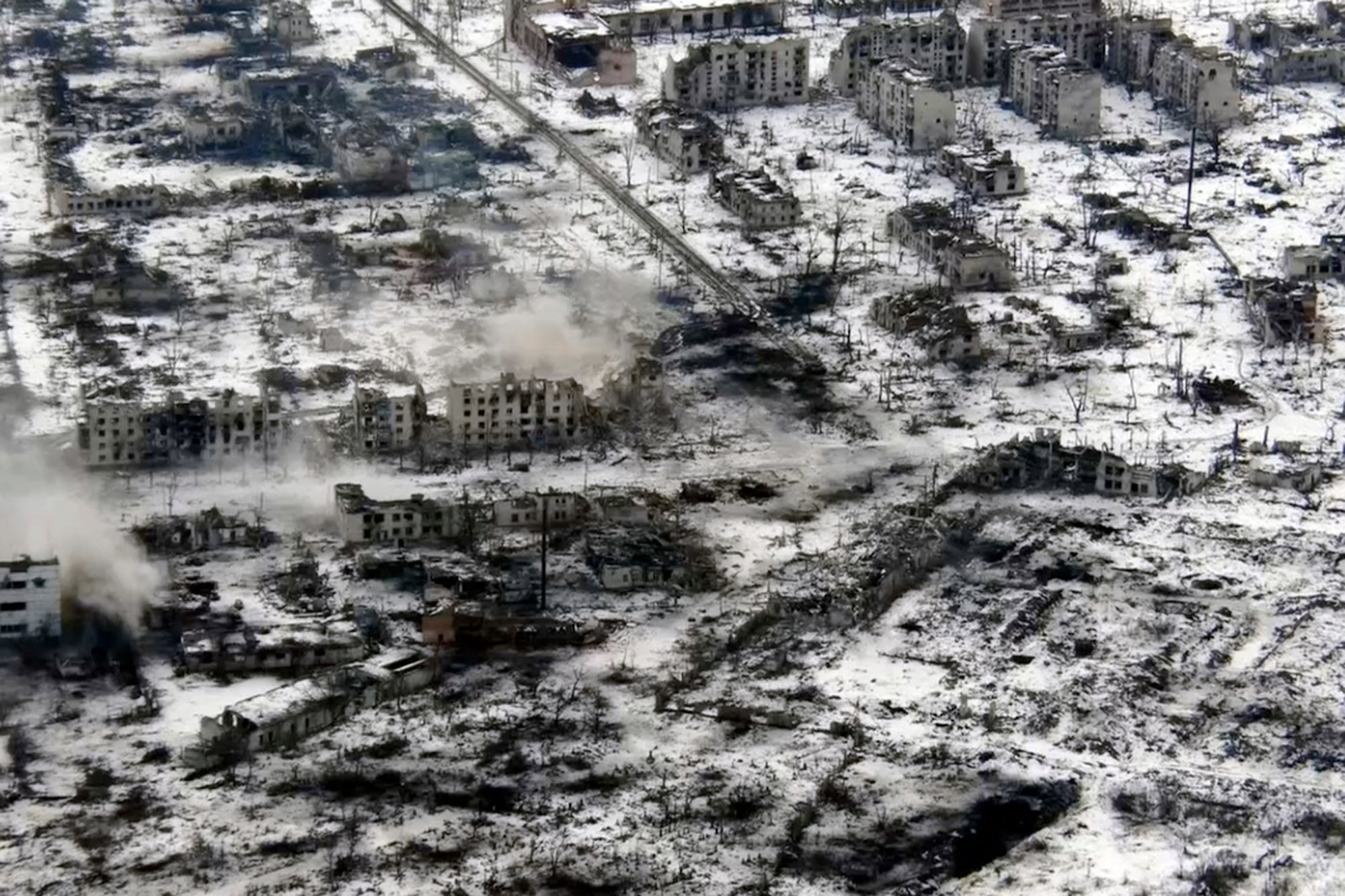This top-down image depicts a desolate town or city in the aftermath of a large-scale destruction, resembling a bombed-out battlefield. The wintry scene is characterized by a predominantly gray and white color palette, with buildings covered in ash juxtaposed against the snow-covered ground. In the lower right corner, there is evidence of foliage amidst the snowy terrain, while more intact structures are seen towards the upper part of the image.

A vertical road runs along the left, dividing the relatively intact buildings from the completely devastated areas where extensive smoke is rising. The foreground is dominated by near-total destruction, with walls and frames of buildings partially standing amidst the ruins, and the highest concentrations of smoke emanating from these areas. Two prominent streets are visible: one runs from the top left into the center, while a perpendicular street cuts across from the middle left to the right of the frame. The lack of observable infrastructure, such as power lines, and the absence of any signs of life further emphasize the town’s abandonment and the severe effects of the armed conflict it has endured.